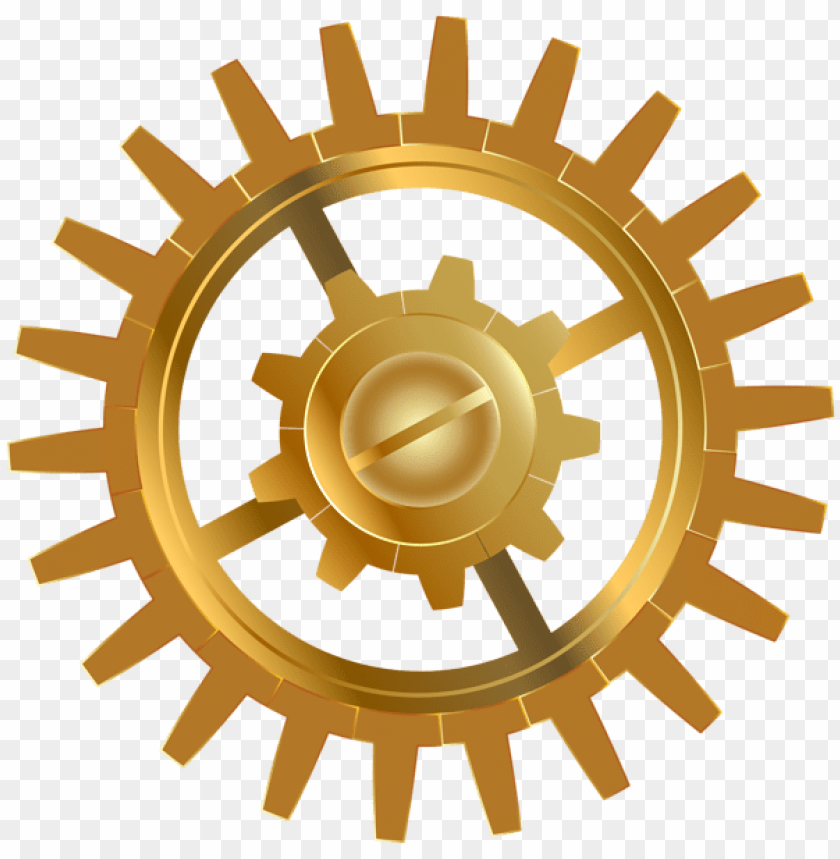This detailed color illustration showcases a gold-colored gear prominently centered within a square format. The gear, depicted with a metallic golden stroke, occupies most of the image from top to bottom and left to right. It features pronounced spokes around its outer edge, allowing it to interlock with other gears. The central part of the gear consists of a smaller circular hub with a crisscross of two long pieces and an affixed screw, designed in the same gold color. Little gears can be seen around the washer behind the screw, adding intricate details to the design. The background is a gray and white checkerboard pattern reminiscent of a transparent layer in graphic software, highlighting that this is a digital rendering or drawing rather than a photograph of an actual object.